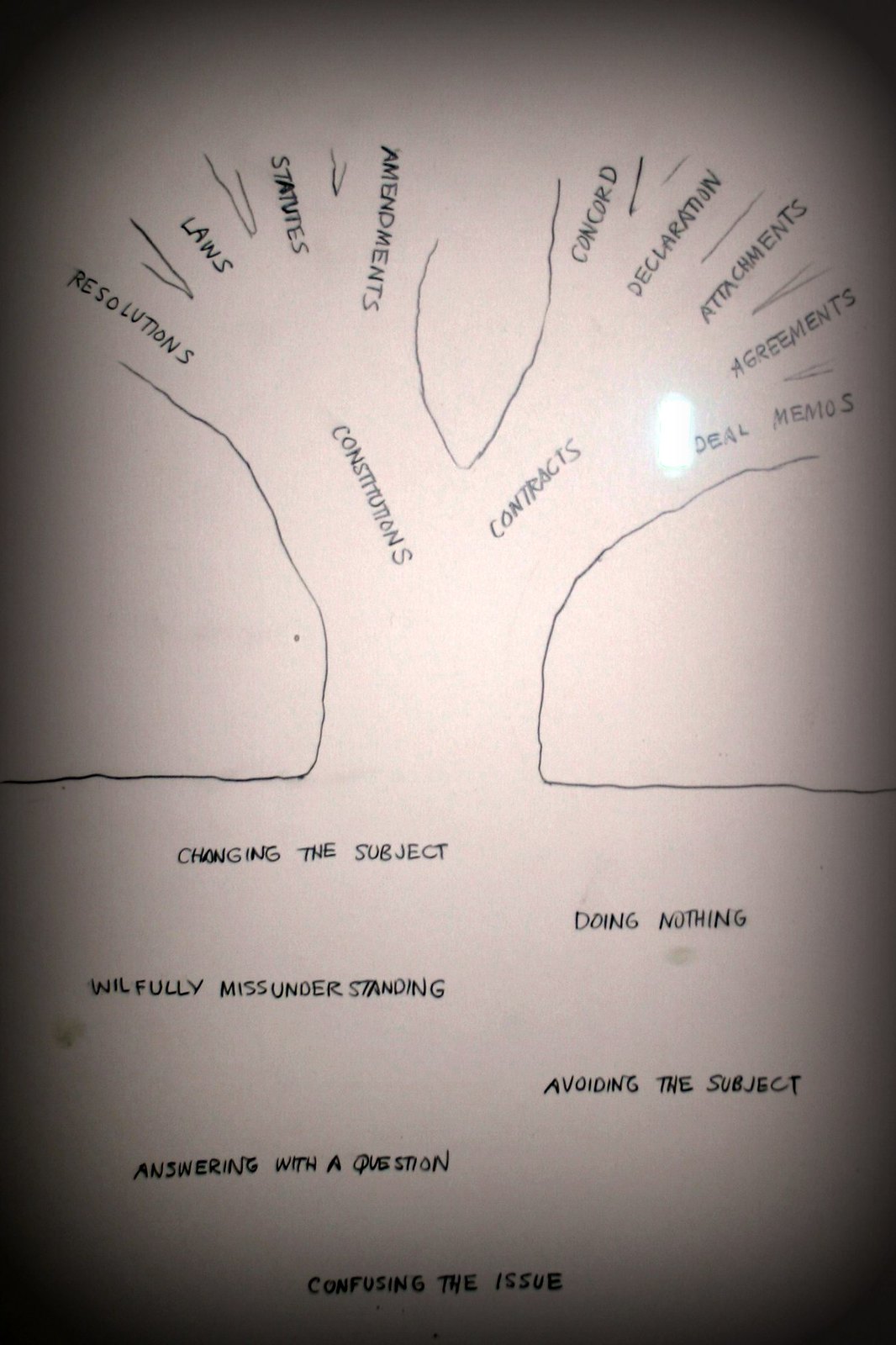The image is a detailed, hand-drawn illustration resembling a tree that may initially appear to be a child’s tracing of hands but has much deeper complexity. This “tree” features two primary branches, labeled “constitutions” and “contracts.” The "constitutions" branch bifurcates into four smaller branches labeled "resolutions," "laws," "statutes," and "amendments." Meanwhile, the "contracts" branch splits into five smaller branches labeled "concord," "declaration," "attachments," "agreements," and "deal memos." Below the tree, mimicking the soil or ground, are phrases such as "changing the subject," "doing nothing," "willfully misunderstanding," "avoiding the subject," "answering with a question," and "confusing the issue." These elements introduce a sense of gravity, suggesting themes tied to historical or instructional content. The image is on a white piece of paper with black corners, suggesting it could be part of a slide presentation, and displays a slight glare, hinting at possible lamination.